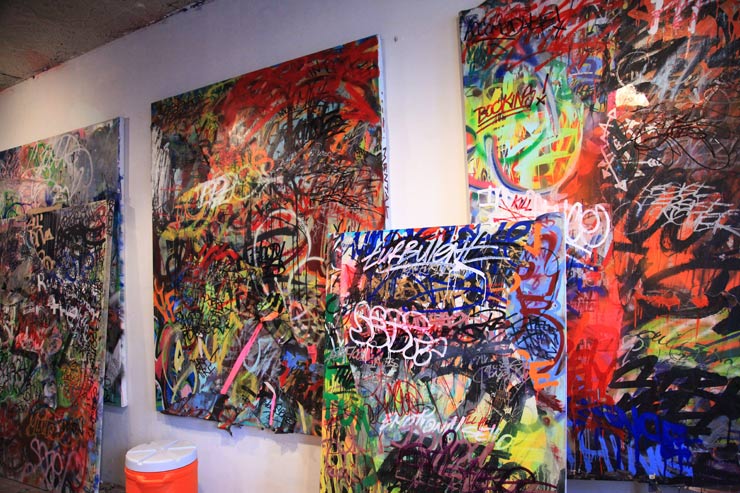This photograph captures a section of an art studio or exhibition, showcasing five vibrant graffiti-style artworks against a plain white wall. Three square canvases are mounted in a row, completely covered in a chaotic tapestry of words, scribbles, and symbols, utilizing nearly every color of the rainbow. Not a single spot of the original canvas remains visible, as each piece is heavily layered with paint, making the writing largely illegible. Among the few decipherable words, "booking!" and "kill" can be seen on the rightmost canvas. On the floor, two additional canvases lean against the ones on the wall; the one on the left rests against the leftmost hanging canvas, while the one on the right is propped up between the remaining two hanging pieces. Completing the scene, an orange Gatorade cooler with a white screw-down lid sits at the bottom left corner, adding a casual, utilitarian element to the otherwise chaotic and colorful display.